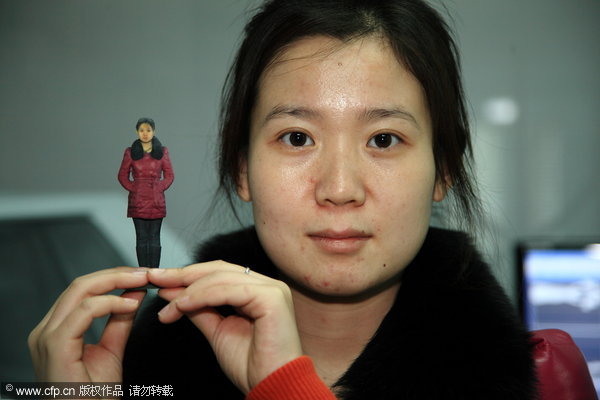This photograph captures an Asian woman with short, dark hair and a slightly freckled complexion, which suggests she may be relatively young. She is dressed in a maroon, thigh-length jacket with a prominent black fur collar. The woman has a bemused expression as she stares straight ahead, appearing amused or curious about the small plastic figurine she is holding in her two hands. This small figurine is a precise replica of herself, complete with the same maroon jacket with a black fur collar and black pants. A ring is noticeable on her middle finger. The background is blurred, but reveals a computer and possibly a television, enhancing the focus on the woman and her miniature counterpart. The only visible text in the image includes some Chinese characters alongside the URL "www.cfp.cn".